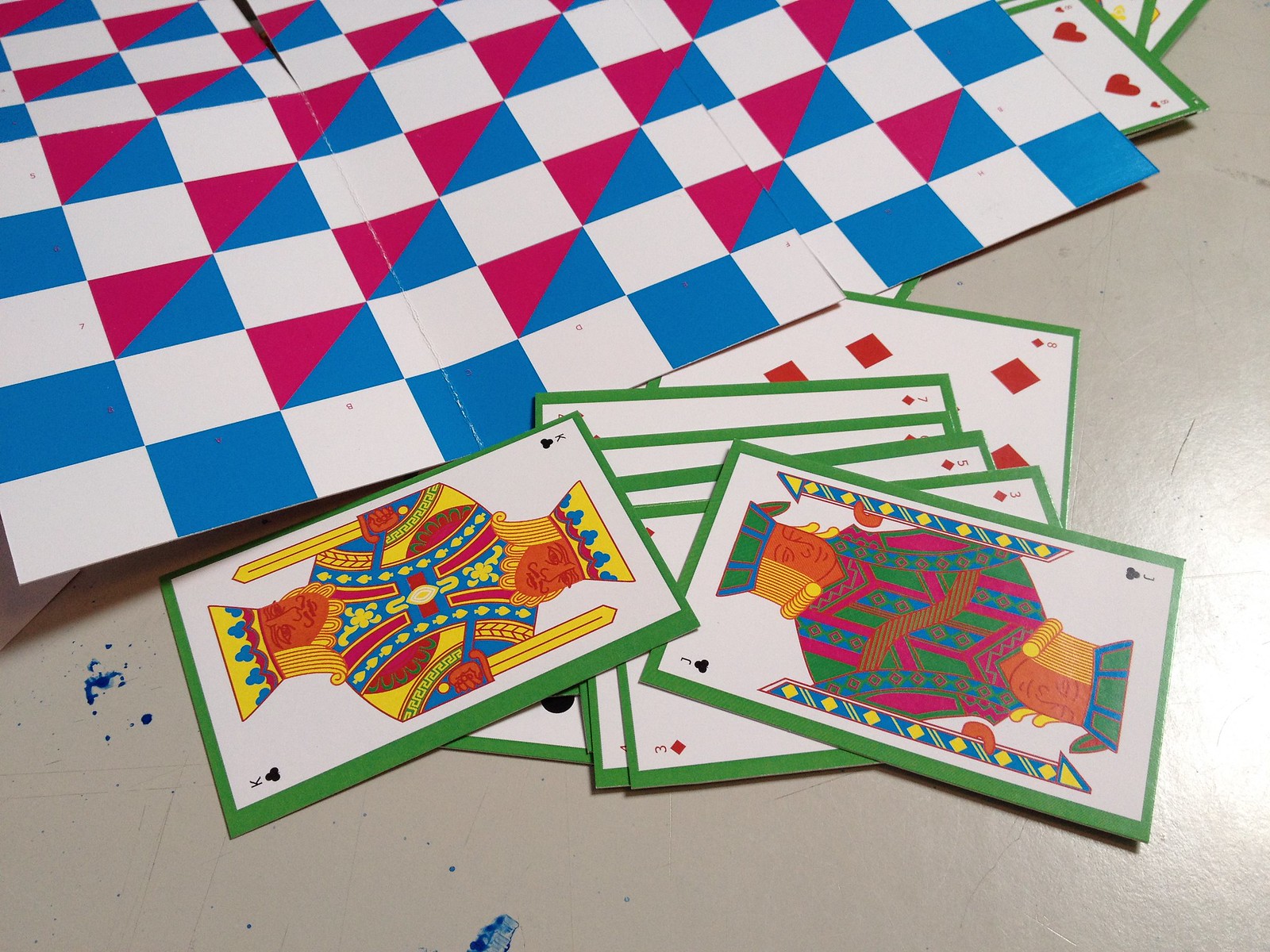The image showcases a scene with scattered playing cards and two thin game boards laid out on a light tan table. The playing cards are slightly larger than standard and include a King and Jack of clubs, both vibrant with an array of bright colors such as yellow, orange, blue, and red on the King, and hot pink, orange, yellow, and blue on the Jack. These cards follow the traditional design where the bust image appears mirrored so that it is always right-side up. Below these cards, partially visible, are additional cards from the deck, including a three of diamonds just beneath the Jack and several other diamond-suited cards. The edges of the cards are bordered in a bright green color.

Adjacent to the playing cards are two game boards, potentially for checkers or chess. The boards seem to be made of a thin material rather than a solid board and feature a pattern of white and blue squares, with some blue squares divided diagonally to include a bright pink triangle. The boards are placed in such a way that one overlaps the other, creating an illusion of misaligned squares. Among the scattered items, another card, the four of hearts, is partially visible under one of the boards. The table itself has a few smudges or drops of blue ink or paint, adding to the eclectic and colorful arrangement.